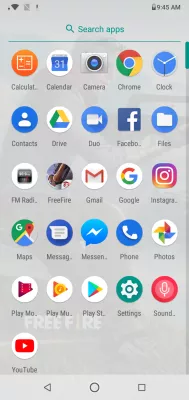This image is a screenshot of a smartphone home screen displaying apps organized in a grid layout. The background is a uniform shade of gray, providing a neutral backdrop for the colorful app icons. There are six rows of app icons, with the first five rows containing five icons each, totaling 25 across these rows. The sixth and final row contains just one icon.

Starting from the top row, the apps are listed as follows: the first app is partially cut off and labeled "Calculate..." which likely denotes the Calculator app. Next to it are the Calendar, Camera, Chrome, and Clock apps.

In the second row, the apps are: Contacts, Drive, an app labeled "Dual," Facebook, and Files.

The third row features: FM Radio, Free Fire, Gmail, Google, and Instagram.

The fourth row consists of: Maps, Messages, Messenger, Phone, and Photos.

The fifth row includes: Play Movies, an app partly labeled as "Play Moo," Play Store, Settings, and Sound.

The sole app in the sixth row is YouTube.

This organized layout of the home screen efficiently categorizes the apps for easy access, showcasing a mix of utility, social media, and entertainment options.